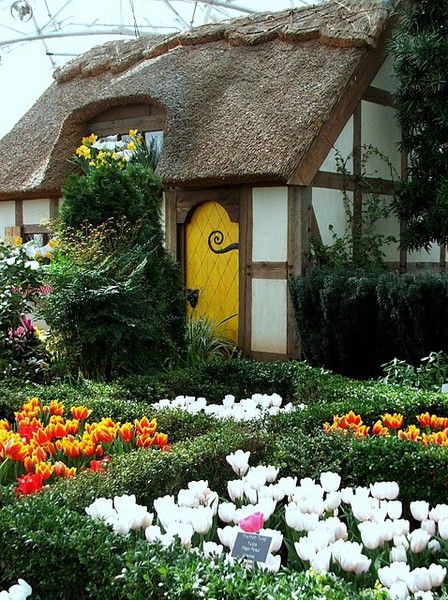This image showcases a charming, fairy-tale-like cottage, reminiscent of old European or Dutch styles. The cottage features a Tudor-style architecture with white wooden walls accented by brown timber, and a distinctive thatched brown roof. A bright yellow door stands out, adorned with curly black cast iron hardware. The cottage is surrounded by a meticulously arranged garden brimming with vivid tulips in a variety of colors: red, yellow, white, and even a few purple ones. These tulips are organized into square flowerbeds, separated by hedges and green bushes. In the lower right corner, white tulips bloom next to a small, gray sign with white writing. To the left and right of the door are patches of red and yellow tulips, with a collection of white tulips directly below the door. Vines begin to climb the cottage walls, adding to its enchanting appeal, while tree branches and a large bush with yellow flowers add a lush backdrop.